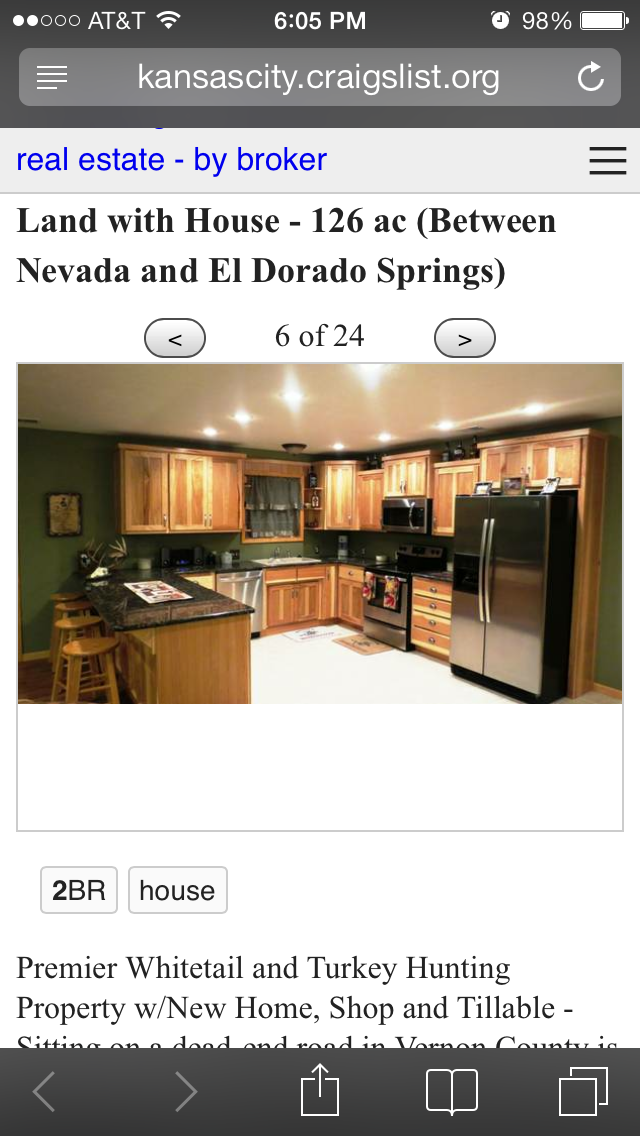The image is a screenshot of someone's cell phone displaying a website, specifically Kansas City Craigslist, under AT&T service with the battery and time indicators visible. The webpage exhibits a listing with a detailed photograph of a modern kitchen. The kitchen features light wooden cabinets with silver handles, a stainless steel refrigerator, an oven with colorful dish towels (red, yellow, and brown) hanging from its stainless steel handle, and a matching stainless steel microwave with a black door. The dark countertops contrast with white cabinetry, complemented by three light wooden stools and a green-painted wall. The kitchen floor is white. Beneath the kitchen photo, the listing text reads: "Premier Whitetail and Turkey Hunting property with new home, shop, and tillable, sitting on a dead-end road in Vernon County" followed by "two-bedroom house." The browser also shows navigation buttons, typical webpage controls, and options to return to the top of the page.